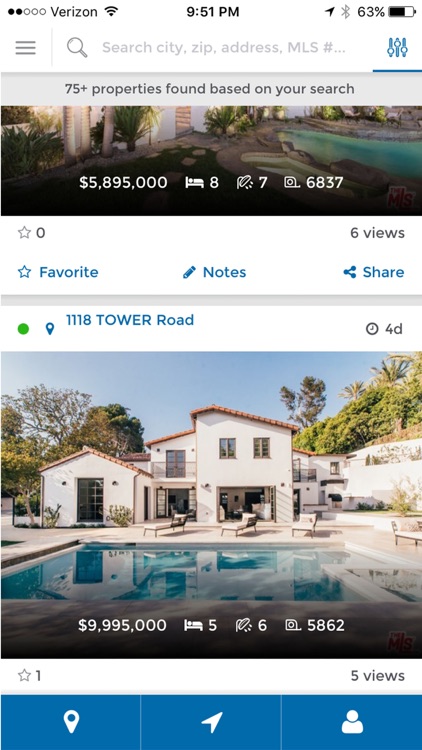A detailed photographic image captures a web search on a mobile device, with various elements displayed clearly on the screen. At the top, two circular bars indicate the Verizon network signal, alongside a Wi-Fi signal icon, showing that the device is connected to a wireless network. The timestamp reads 9:51 PM. Situated at the very top is the location bar, showing that the Bluetooth is switched off, as indicated by the grayed-out icon, while the battery life stands at 63%.

Below these indicators, a prominent white search bar is visible, equipped with a magnifying glass icon and placeholders for searching city, ZIP code, address, or MLS number. Next to the search bar, a blue "Filters" option is present.

The main part of the screen showcases a brightly colored real estate listing. The image reveals a luxurious property labeled with a staggering price of $505,895,000. This property appears to accommodate eight people and includes seven bathrooms. An icon resembling a camera is also present. In the image, a pool and lush foliage are clearly visible.

Towards the bottom of the screen, another complete property listing for 1118 Tower Road is displayed. This listing features a white house with a slanted roof and a visible pool, priced at $9.995 million.